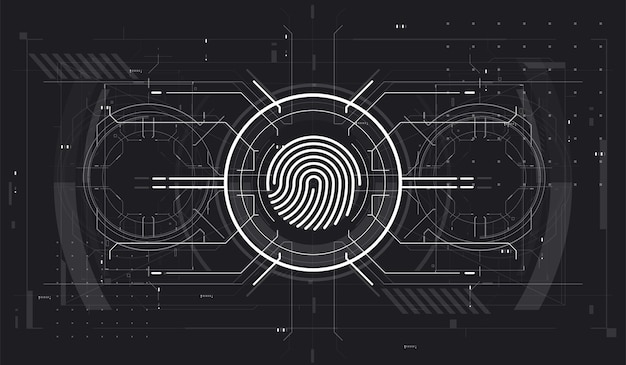This is a rectangular diagram set against a black background, featuring a prominent white circle at its center. The central circle contains intricate, swirled lines resembling a fingerprint. Surrounding this primary circle is a thinner white ring. From the central motif, various lines extend in different directions. Flanking it on both the right and left are additional lighter white circles, each connected to the main circle by two parallel lines. These side circles are adorned with smaller dots and lines that form half-circle, concentric, and radiating patterns. Additional elements, including series of dots forming an 8x7 grid and numerous lines in white and gray, are scattered across the diagram, lending a blueprint-like aesthetic. Overall, the image conjures a sense of both technological and schematic design.